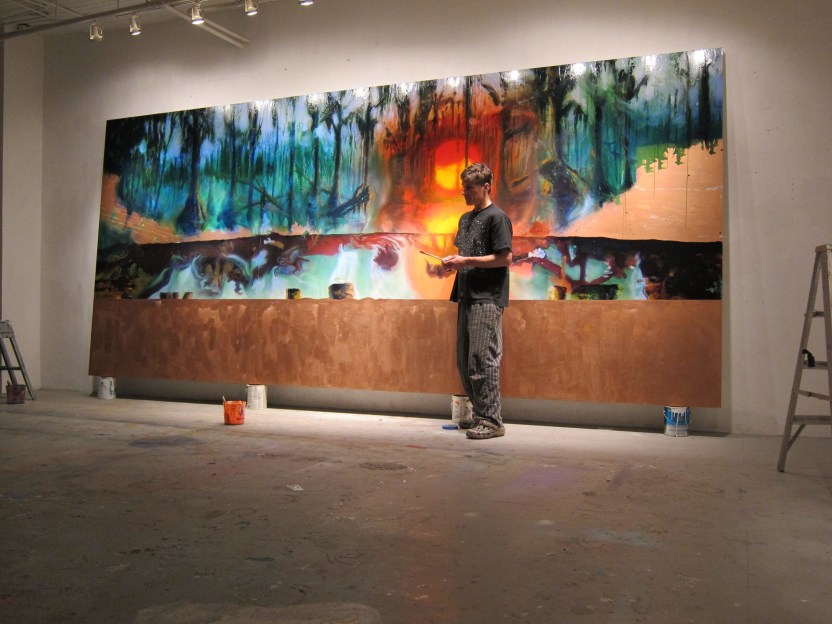In a brightly lit art studio, a fair-skinned man with a bowl-cut hairstyle, dressed in a black t-shirt and comfy baggy striped brown-and-dark-brown pants, stands before a colossal mural-style painting that towers two feet above him and stretches between 20 to 30 feet across. The painting, propped up on four paint cans positioned at its quarters, appears half-completed. The top half bursts with color, depicting a vibrant sunset with a reddish-orange sun peeking through long, thick black trees with green foliage, while shades of red, blue, white, black, green, and various browns add depth. The center features a serene lake reflecting the sun and trees above. In contrast, the bottom half remains bare, showing only light brown, canvas-like brush strokes. The floor around him is cluttered with several paint containers, including visible white and orange paints, indicating the ongoing creative process.